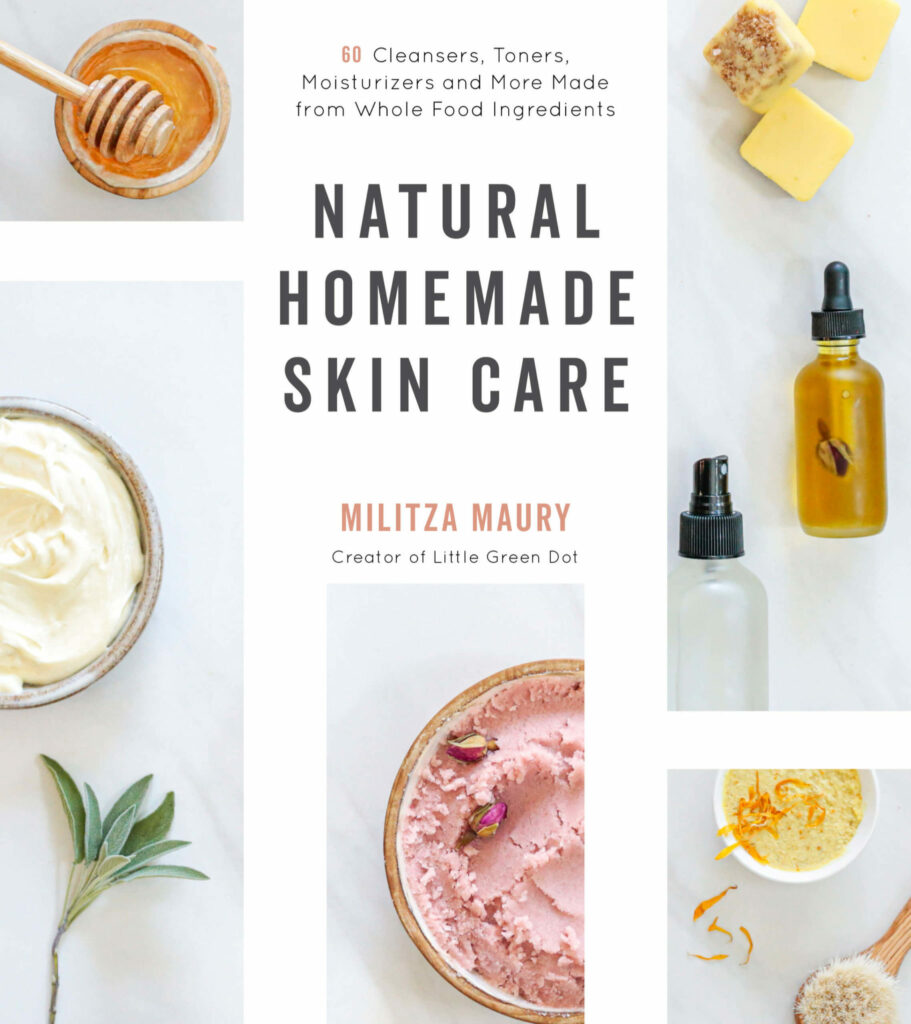The image depicts the cover of a book with a white background, featuring a collage of various natural elements and containers. At the top, the text in black reads, "60 cleansers, toners, moisturizers, and more made from whole food ingredients." The focal point in the center highlights in bold, "Natural Homemade Skincare," authored by Melissa Militza, creator of Little Green Dot. The collage includes a wooden honey stirrer in a glass of honey in the upper left corner, a gray bowl containing white cream with a sage leaf beneath it, and a bowl of pink cream or material in the middle. The right side showcases two vials, including a spray bottle with a black top and golden liquid, as well as pieces of what appears to be white cheese. Additionally, there are some butter cubes and a brush in the bottom right corner. This cover effectively combines various natural ingredients, emphasizing the use of whole food components in DIY skincare products.